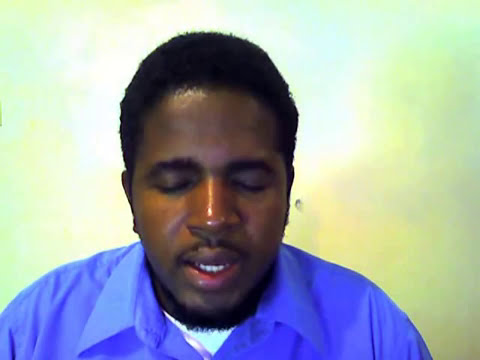The image depicts an African American man, likely in his mid to late 20s, with short black hair, a black beard, and a black mustache. His eyes are closed, and his mouth is slightly open, suggesting he might be in the midst of a prayer or speaking. He is wearing a blue, collared button-up shirt with a white t-shirt underneath. The background appears to be a mix of light green, yellow, and white, with a pixelated quality indicating it was taken with a low-quality camera. There is a noticeable shine on his prominently featured nose, and the lighting creates a shadow that casts onto him. The man's head is centered in the frame, with his shoulders and chest partially visible at the bottom.